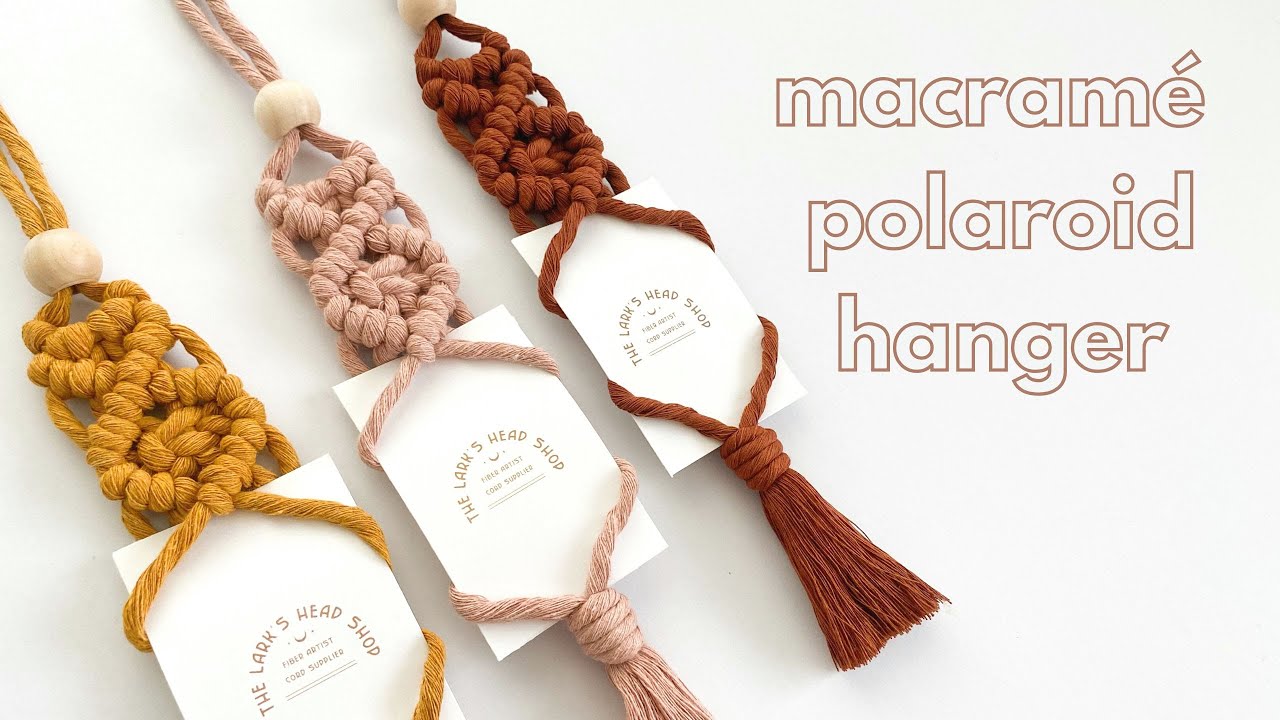The photograph showcases three intricately braided macrame hangers on a white background, each holding a piece of paper inscribed with "The Lark's Head Shop." To the right top corner, text in a brown outline reads "Macrame Polaroid Hanger." There are three hangers aligned diagonally from top left to bottom right. The first hanger on the left is a golden yellow or orangish-yellow color, the middle one is pink, and the one on the far right is a reddish-brown. Each macrame hanger is crafted from fabric braided together, forming a flat, rectangular shape with diamond patterns and ending in tassels. They also feature macrame tying at the top and wrap around the white card that appears to have additional unreadable text, possibly an address or a phone number.